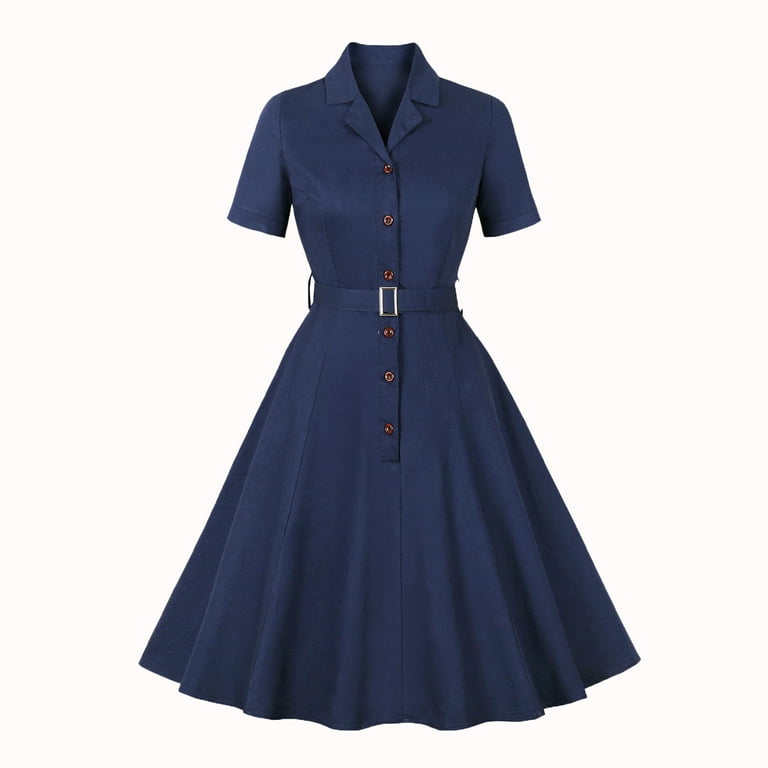This product photograph showcases a vintage-style women's shirt dress designed for both formal and casual occasions. The dress is crafted from dark navy blue fabric, resembling denim but is not actually made from denim. It features a standard shirt collar and short, fitted sleeves that add a touch of elegance. Running down the front are six dark brown buttons, extending from the collar to just below the knee, emphasizing its button-up style. The waist is cinched with a matching navy blue belt, complete with denim belt loops and a prominent silver buckle. The top of the dress is form-fitting, while the skirt flares out to a full, flattering shape. The background of the image is entirely white, devoid of any distractions, making the dress the focal point.